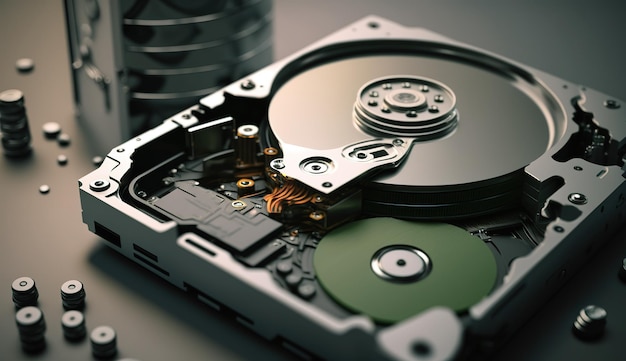This photograph captures the intricate interior of what appears to be a disassembled CD-ROM or DVD player, showcasing the detailed components and mechanical structure within. At the center of the image, there is a prominent square-shaped metal frame featuring a large circular section on the right side, reminiscent of where a CD would be placed and rotated. This circular part has a small gear in the middle and is connected by orange wires, which suggests its function as part of the disc reading mechanism. Nearby, on the left side, there's a smaller sage green disc with a central circle, which is possibly part of the electronic control system. Five bolts are visible on the bottom left corner, securing some sections of the device, and scattered around are other small, round objects that might be screws or additional components. In the background, blurred and out of focus, is another metallic piece of equipment, adding to the workshop-like setting where this delicate machinery is being examined or repaired.